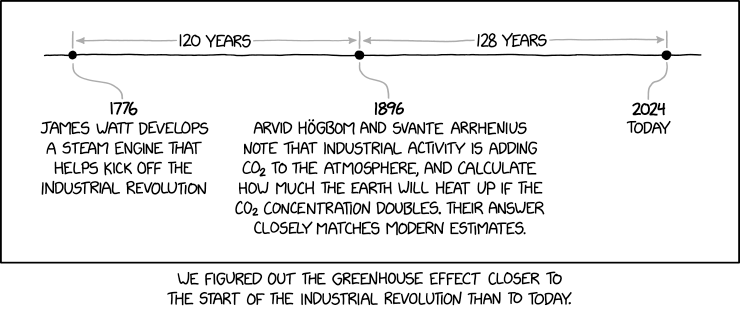The image features a long horizontal rectangle outlined in black with a white background. Across the center of the rectangle runs a horizontal line, punctuated by three dots: one at the beginning, one at the middle, and one at the end.

- At the first dot on the left side, a grey line leads downwards to the text: "1776, James Watt developed a steam engine that helped kick off the Industrial Revolution."
- The middle dot has another grey line beneath it leading to the text: "1896, Arvid Högbom and Svante Arrhenius note that industrial activity is adding CO2 to the atmosphere and calculate how much the Earth will heat up if CO2 concentration doubles. Their answer closely matches modern estimates."
- The final dot on the right is linked to the text: "2024, today."

Above the first and middle dots, the text "120 years" is displayed in black with grey arrows pointing outwards on both sides. Similarly, between the middle dot and the right dot, the text "128 years" is displayed with grey arrows pointing outward on both sides.

Below the entire rectangle, outside of the outlined area, a cartoonish, comic sans-like font reads: "We figured out the greenhouse effect closer to the start of the Industrial Revolution than today."

This detailed caption effectively conveys the historical timeline presented in the image, highlighting key milestones in the understanding of climate science.